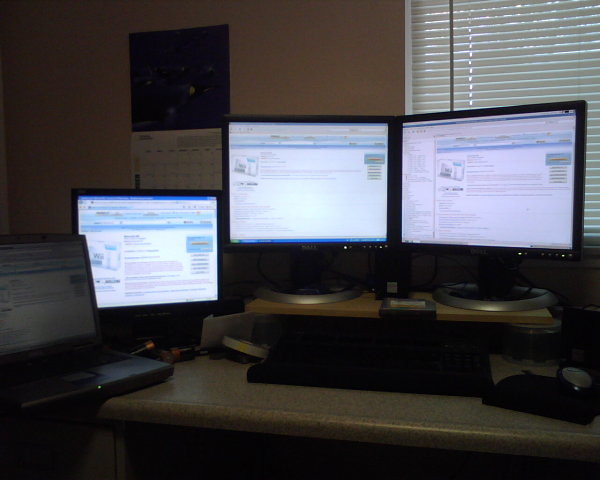In this photograph taken inside a dimly lit study or home office, likely at night, a desk made of pale pine wood houses a black laptop and three additional monitors, making a total of four lit screens. Two of the monitors are elevated on a matching wooden stand, with a keyboard and mouse situated underneath. The wall behind the setup is a beige color, featuring a wall calendar in the top left corner whose image and month are obscured due to poor lighting. In the top right corner, a window with horizontal blinds drawn shut blocks out any natural light. Despite the overall darkness of the room, the screens illuminate the immediate surroundings with a soft glow, displaying what appears to be text, possibly from a browser or Wikipedia.